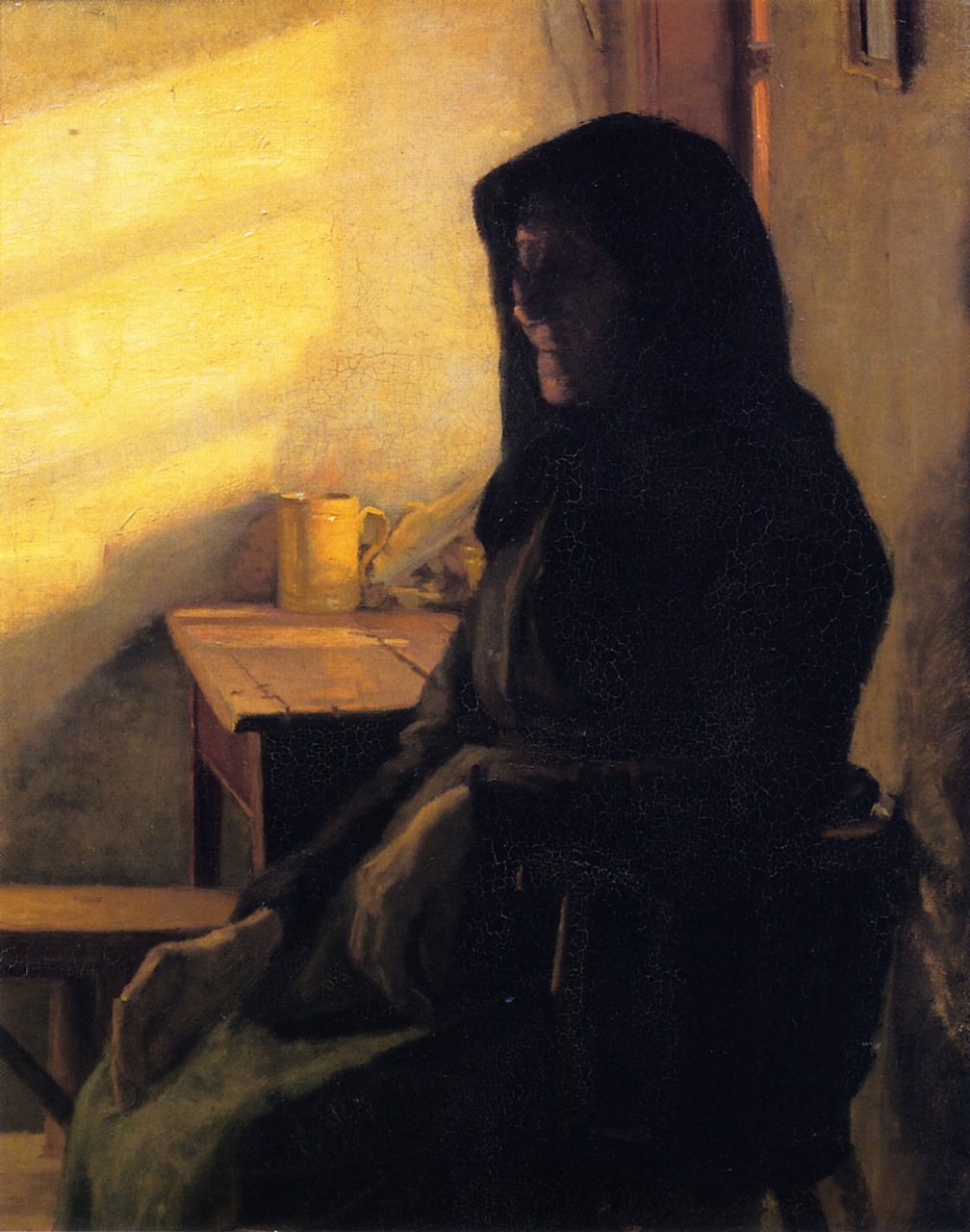This artwork, titled "A Blind Woman," is a vertically aligned rectangular painting depicting an elderly woman seated against a wall on the right side of the image. The woman, who appears to be sleeping, faces toward the left with her head slightly bowed. She is clad in a dark hooded robe or shawl that drapes over her shoulders and down her back, adding a sense of weight and solemnity to her presence. Her wrinkled face and hands—one resting limply on her lap and the other hanging off the armrest of a wooden barrel-style chair—suggest a life marked by age and possibly struggle. 

To the woman's right, positioned in the middle of the image, stands an old wooden desk adorned with yellow splashes and a yellow metal pitcher dripping something brown. The desk, a matching wooden stool beneath it, and a shadowy, almost black lower half of the wall behind them evoke a rustic, worn-down environment. Light filters into the dim room, casting yellow panes on the yellowish-brown, cracked walls, hinting at a window blocked by the woman's figure. Above her head, a small framed picture or mirror hangs, its details obscured except for a grayish interior.

The overall scene is pervaded by a melancholic tranquility, highlighting not just the solitary woman but also the passage of time etched into every surface around her.